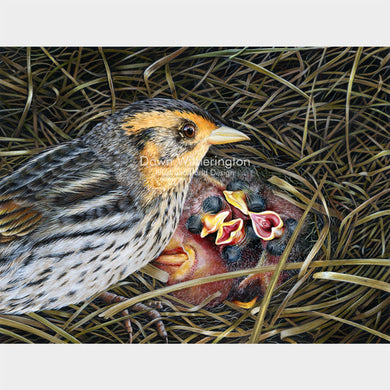This square photograph features a striking scene of a mother bird and her four newborn chicks nestled in a circular, straw-like nest composed of light brown, wispy material. The top and bottom of the image are framed by light gray bars, indicating either an effect or a possible screenshot from a video. In the center of the photo, there is a barely legible, light gray watermark, possibly reading "David Witherington," presumably the name of the photographer.

The adult bird, perched prominently on the left side of the nest, displays a vivid profile marked by a combination of orange and black feathers. Her face is adorned with orange feathers, transitioning to a black forehead and brown eyes circled by black. The side of her head appears goldish or yellowish. Her wings and back feature intricate black and white stripes and dots, while her belly is primarily white with subtle black speckles. The mother bird has a light orange beak, adding to her striking appearance.

Centered within the nest lie four very young chicks, their pinkish, featherless bodies contrasting sharply with their orange beaks and black, closed eyes. Two of the chicks have their mouths open, revealing the red interiors. The surrounding background is filled with thin, light brown pieces of grass, seamlessly blending with the nest. The photograph captures an intimate moment in the life of these birds, emphasizing the care and presence of the mother alongside her fragile, dependent offspring.